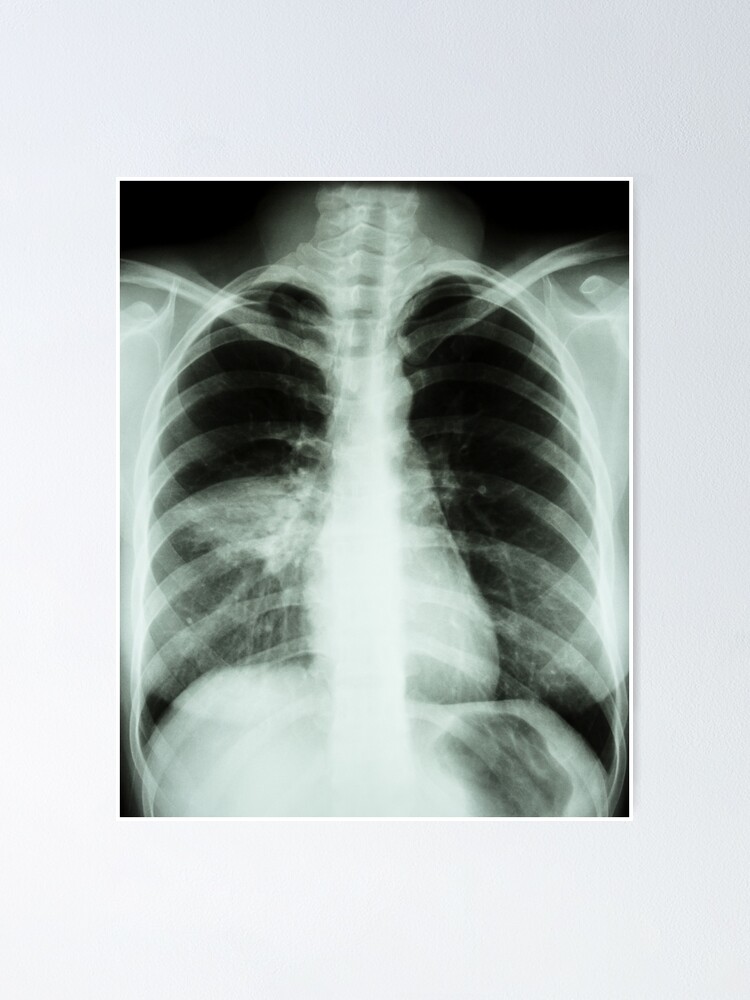This detailed image is a black and white x-ray of an adult's chest, displaying a front view. The x-ray vividly captures the rib cage and the prominent bones of the shoulders and arms, tapering down to include a portion of the pelvis. The spinal column, slightly inclined towards the right, is faintly visible, along with the collarbones. The lungs appear dark within the central cavity, with the right lung showing some opacities towards the base. The heart is discernible in the middle, maintaining a normal contour and occupying approximately half of the chest's width. The ribs exhibit a white chalky appearance with some hazy fuzziness. The background is predominantly black, contrasting with the highlighted skeletal structure. Notably, there are white masses along the spine and a possible white clouded area in the left lung, suggesting potential abnormalities. The rectangular image extends from the mid-neck down past the ribs, providing a comprehensive view of the chest cavity. There is no text or date visible to provide further context about the x-ray.